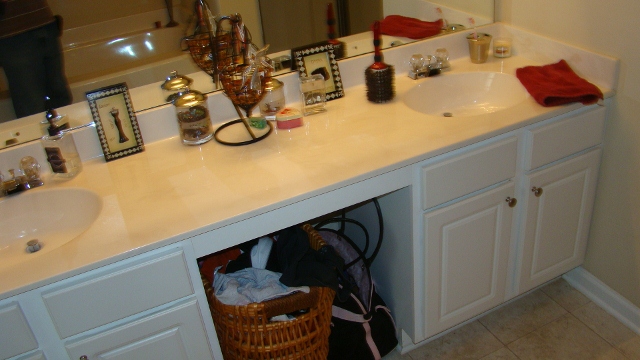The image is a first-person POV shot of a bathroom sink area. The countertop, cabinets, and sinks are all white, presenting a bright and clean aesthetic. There are two sinks on the tabletop—one positioned on the far right and the other on the far left. Below each sink, there are two vertically-aligned rectangular cabinets. Both sets of cabinets feature gold circular handles, with the left-side cabinet handles positioned in the top right corner and the right-side cabinet handles in the top left corner.

Above the sinks and countertop, a large mirror spans the wall, capturing the reflection of the person taking the photo. The individual is wearing denim jeans and a brown and white striped shirt, visible in the top left corner of the image. Behind this person, the mirror also reflects a simple white bathtub.

On the countertop, there are a few items arranged. Next to the left sink, a hairbrush lies close to the right edge. Additionally, there is a red towel and a golden cup in the right corner of the bench, which holds a toothbrush. The overall scene captures a neat and tidy bathroom setup with thoughtful attention to detail.